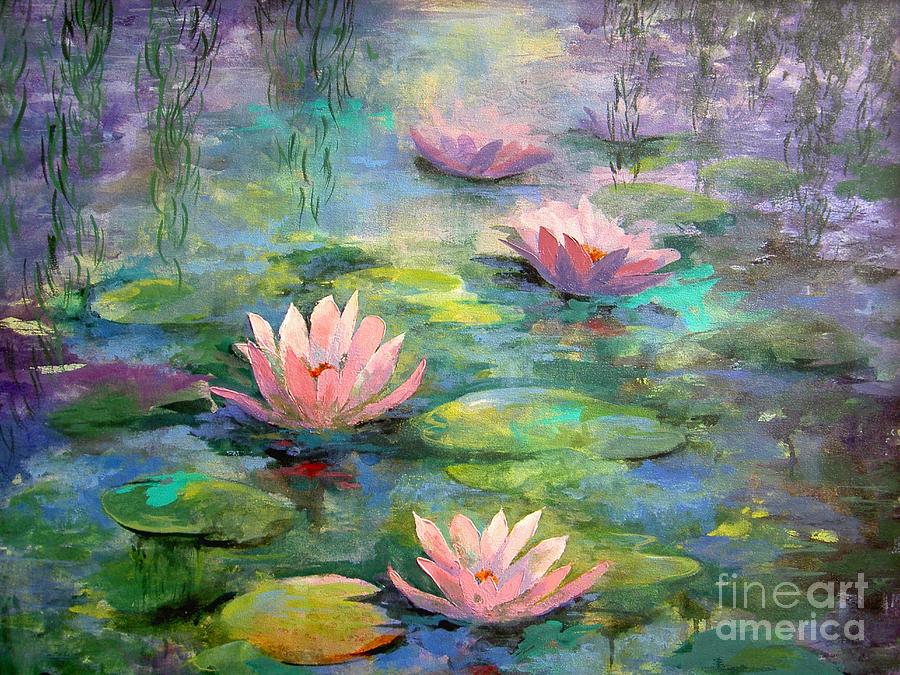This image depicts a serene acrylic painting, oriented in landscape format, measuring approximately six inches wide by four inches tall. At the bottom right of the painting, the watermark "Fine Art America" is inscribed in a light gray, almost translucent print. The scene captures a tranquil lake adorned with vibrant water lilies and lily pads. The flowers themselves, predominantly pink and purple, transition in hue as they recede toward the horizon. The water reflects these colors, creating a gradient from blue and teal to purple, evoking the impression of a sunset.

Towards the center, the water is painted in various shades of blues and greens, infused with an array of colors including yellow, black, and teal, making the surface appear dynamic and lively. Green and yellowish lily pads float atop the water, with some displaying large blooming flowers that incorporate pinks, purples, creams, and whites. Scattered amid these are delicate green leaves and strands of green vines, which cascade from the upper corners of the painting, resembling willow leaves. The artwork conveys a soft texture throughout, enhancing its tranquil and picturesque quality.